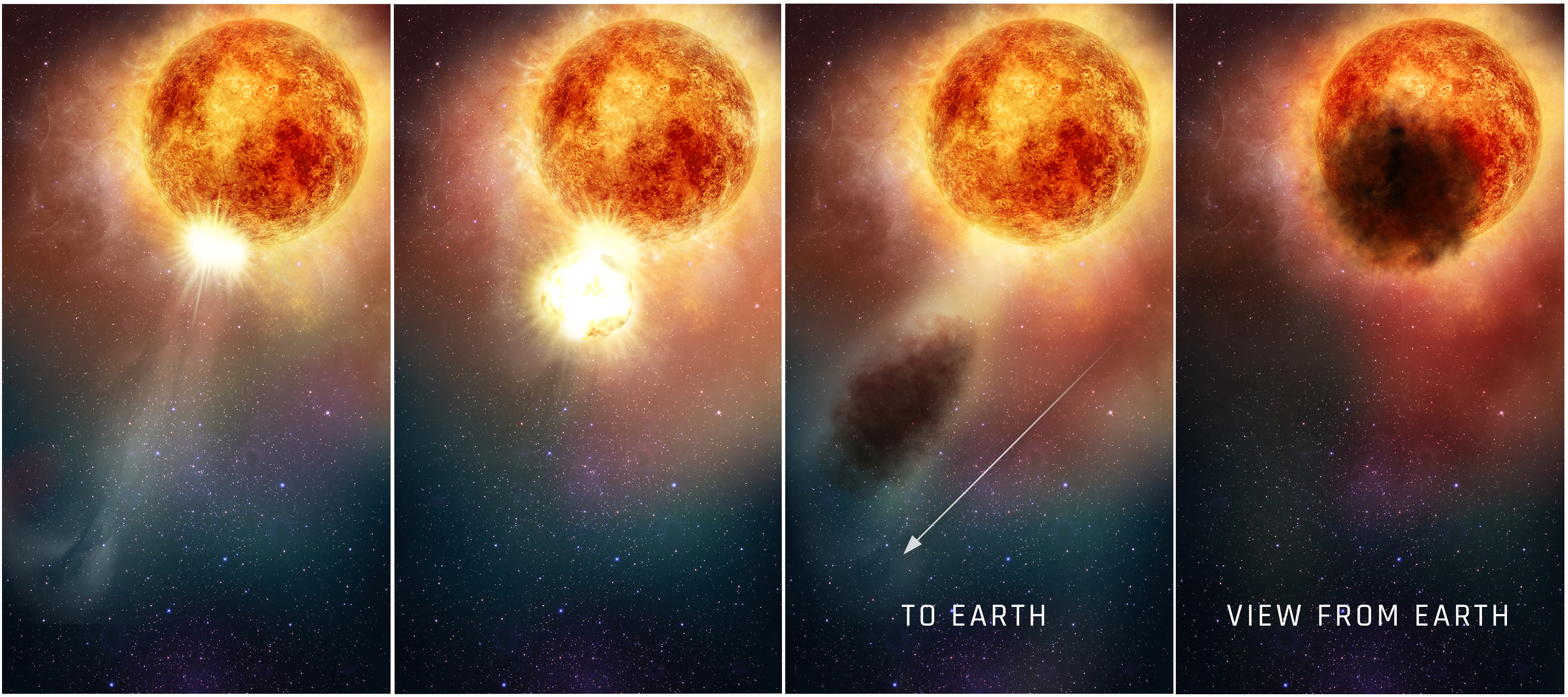A series of four successive images portray a cosmic event involving the Sun. In the first image, positioned in the upper right, the Sun is depicted with bright and vibrant rays emanating from its surface, with a small white object, possibly a star, asteroid, or planet, situated below. Stars twinkle subtly in the background. In the second image, the Sun is closer, and the emanating rays have expanded significantly, suggesting a growing solar flare or an erupting particulate stream. The third image shows a further evolved state where the flare has spread more widely. An arrow points from the right middle of the frame down to the bottom left, labeled "to Earth," indicating the direction of the cosmic stream. By the fourth image, the flare or particulate cloud has obscured a substantial part of the Sun. This obscuration creates a dramatic dark mass against the Sun, which is labeled "view from Earth." The vibrant hues of bright oranges and reds provide a stark contrast in each image, enhancing the visual representation of the celestial phenomenon.